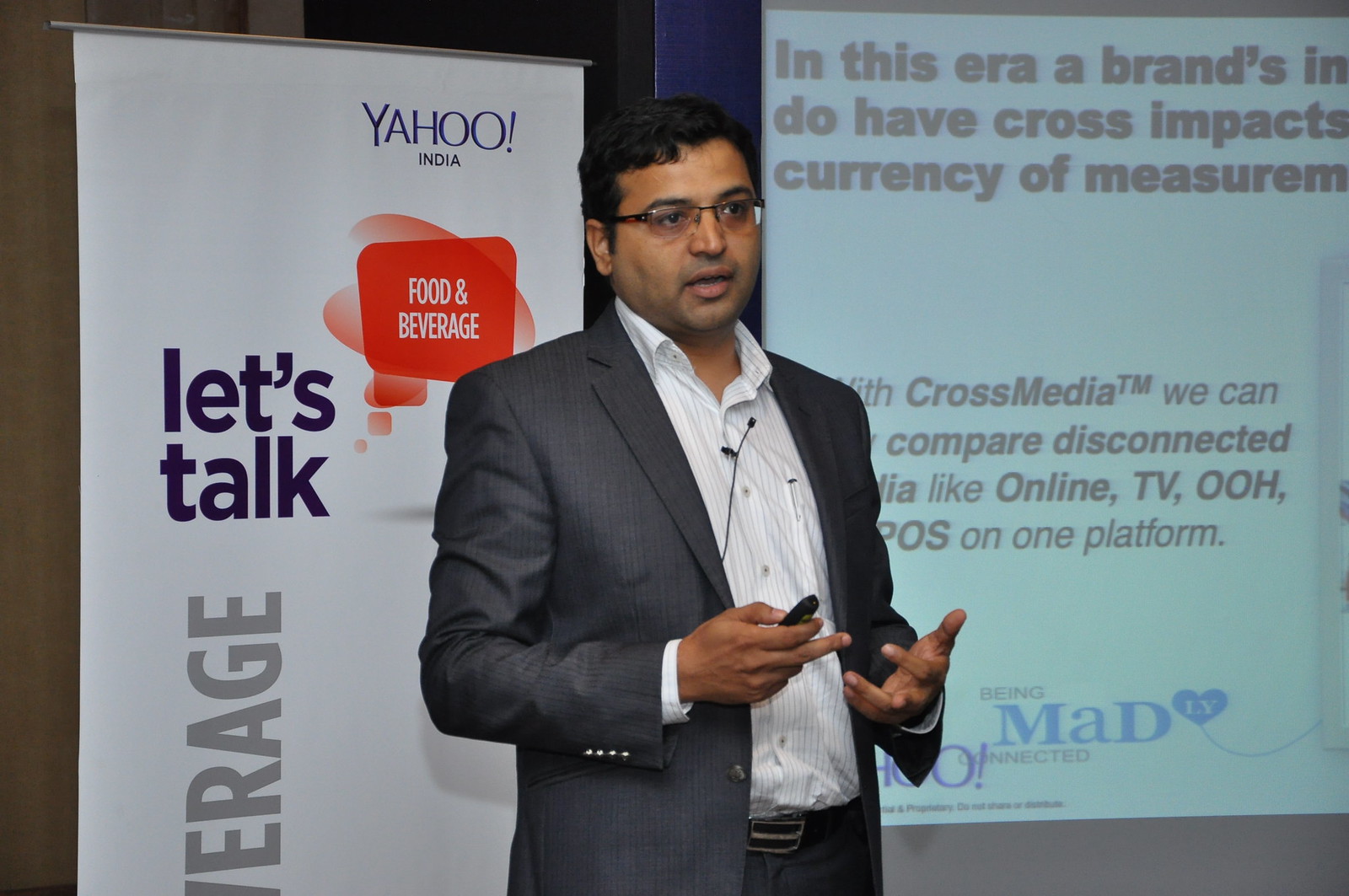The image features a man of likely Indian descent, giving a presentation at what appears to be a conference. He is standing at the center of the image, facing the camera. The man has black hair, glasses, and caramel-colored skin. His attire includes a gray suit jacket paired with matching gray pants and a white button-down shirt without a tie. A black microphone is pinned to his shirt, and he holds a black clicker in his right hand, gesturing expressively as he speaks.

Behind him, a vertical banner prominently displays the text “Yahoo India” in large letters, along with “Food and Beverage” and “Let’s Talk” in colorful sections (red, purple, blue, and gray). To the left of the banner, a projector screen shows a slide featuring partially visible text about cross-media comparisons: "In this era, a brand's [...] do have cross impacts [...] currency of measurement [...] With cross media we can compare disconnected media like online, TV, OOH, POS on one platform."

The setting appears to be a professional environment, likely a conference or seminar, where the speaker is addressing the audience on media strategies or related topics. The composition and colors in the image contribute to a formal, business-like atmosphere.